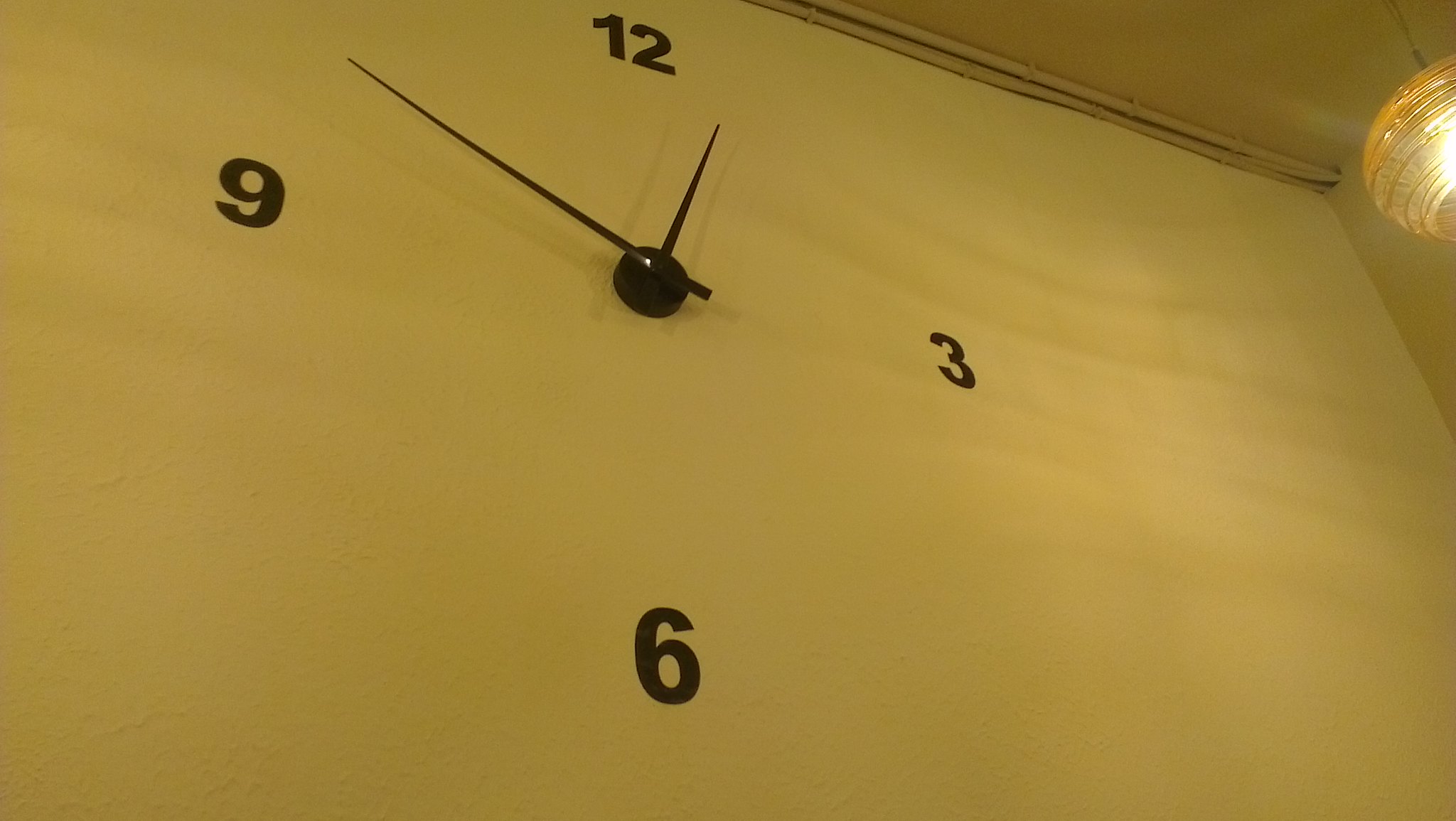The image showcases a minimalist clock embedded into a pristine white wall. Positioned in the upper right corner of the frame is an illuminated globe light fixture, notable for its open-bottom design. The clock itself is starkly simple, displaying only the numbers 12, 3, 6, and 9 in black. The clock's hands and the central knob anchoring them are also black, contrasting sharply against the white backdrop. Lacking additional numbers or tick marks, the time appears to be approximately 12:50.